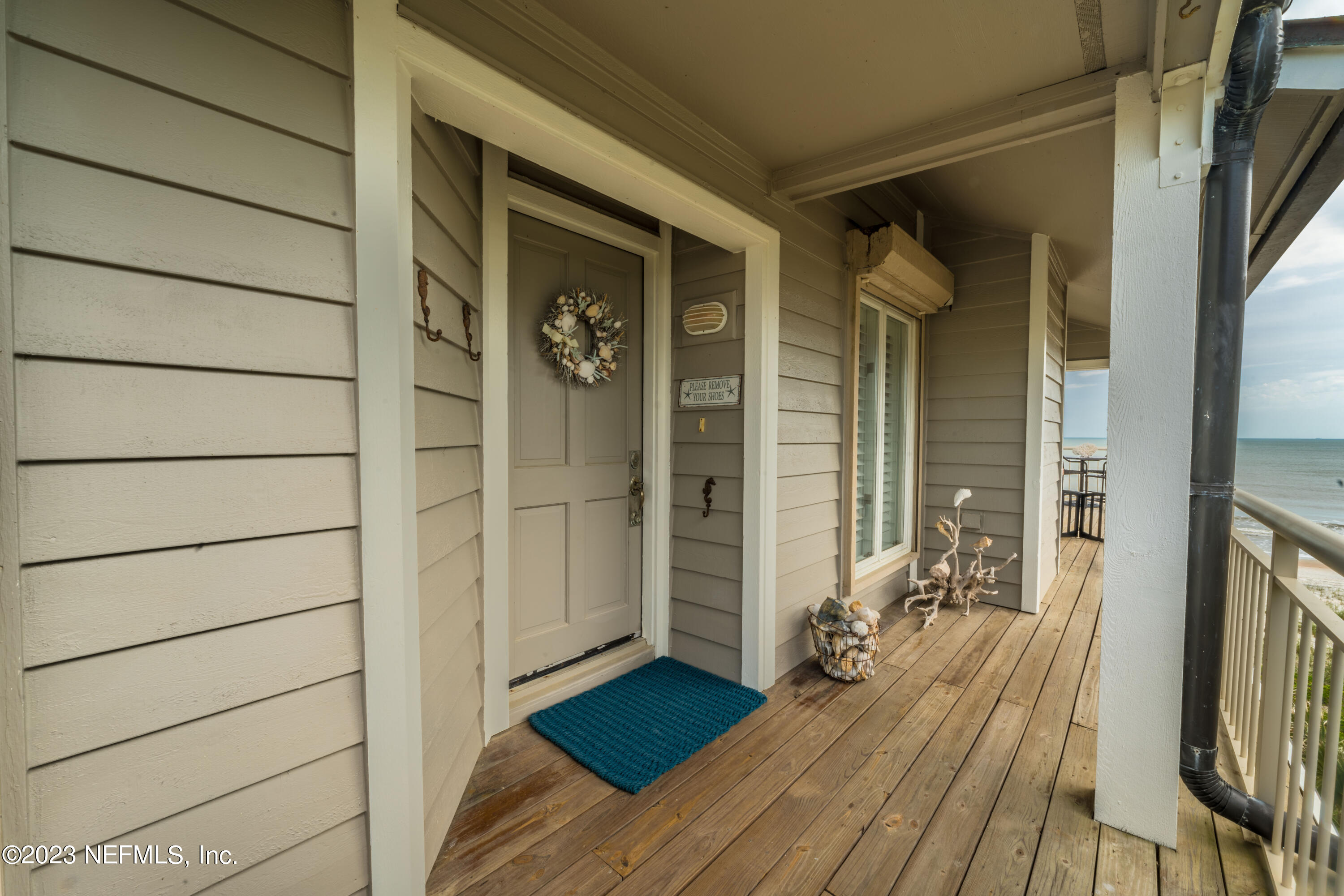The image captures the front porch of a beige-toned beach house, with light brown wood decking and white railing. The house features coastal decor, including a seahorse-shaped hooks and a reef-themed wreath hanging on a beige door. In front of the door lies a vibrant blue welcome mat. The porch showcases various maritime-themed ornaments, like a basket of seashells and a piece of driftwood adorned with more shells. Visible elements around the porch include a white column, black gutter, and a nautical-style light fixture. A large white window sits alongside the door, beneath which a mini-split air conditioning unit can be seen. The scene is complemented by the expansive view of a greenish hue ocean and cloud-covered sky in the background, with a sliver of sandy beach. The bottom left corner of the photograph is watermarked with "Copyright 2023 NEFMLS Inc."